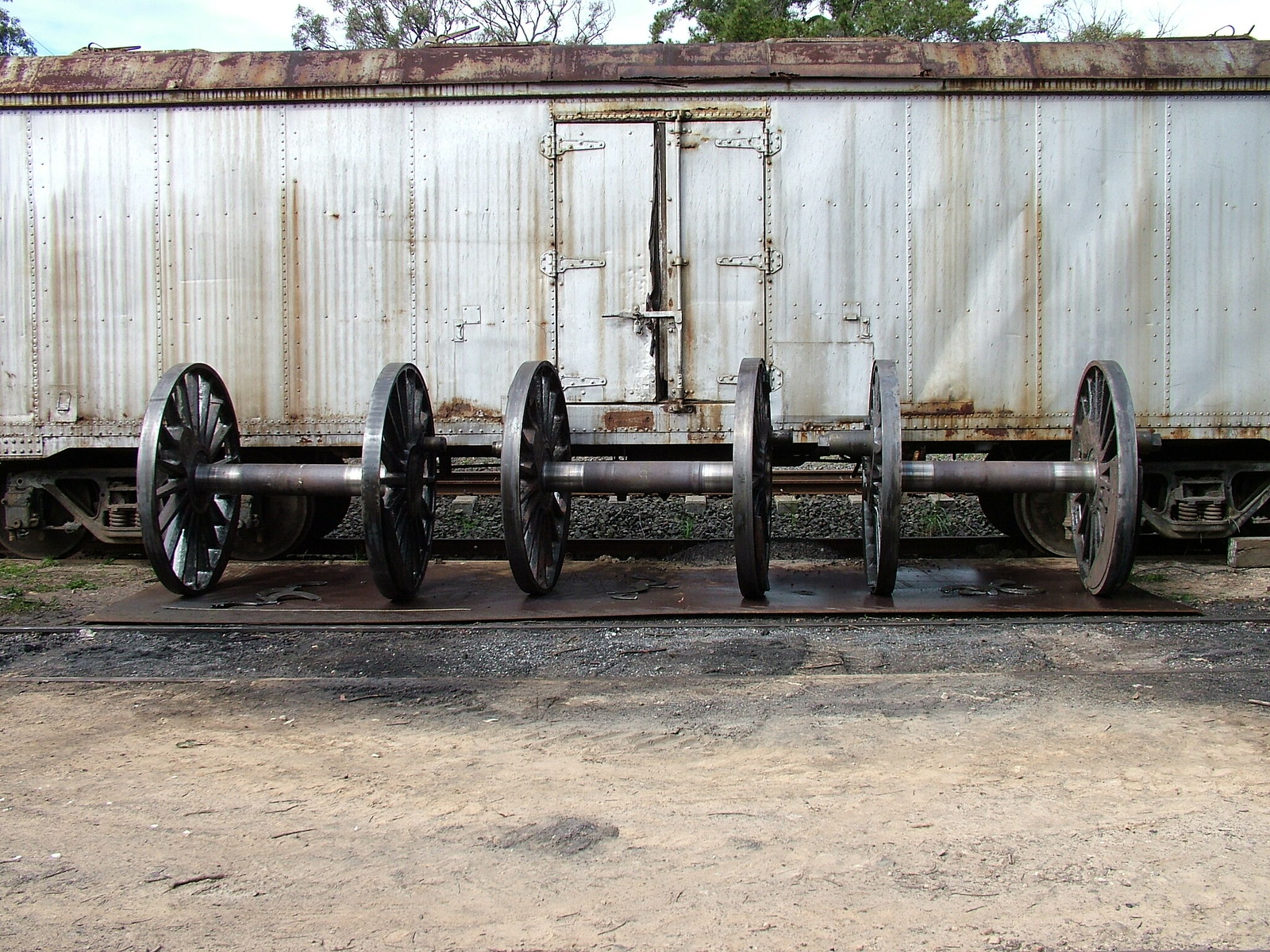In the photograph, an old and weathered rail car fills the width of the image. The car, an off-white color heavily rusted and stained with vertical brown streaks from water runoff, has steel walls and doors alongside an iron roof, all showing signs of extensive rust. Its central door features a latch and sits prominently on the car's side. The rail car rests on browned, blackened dirt, reminiscent of a typical rail yard ground.

In front of the train car, three large pairs of metal wheels, each mounted on separate axles, are laid out perpendicular to the rail car. These wheels, which are equipped with a crank device on one end, appear to be designed for train tracks and are situated on a large metal sheet, likely to prevent them from sinking into the loose dirt below. Surrounding the wheels and train car, the foreground features a mix of blackened and regular brown dirt, with some tire tracks indicating recent movement.

Behind the rail car, a rocky embankment is visible along with sparse vegetation, including a few small plants and scattered trees. The scene is set against a backdrop of these elements, suggesting an abandoned or less maintained section of a rail yard.